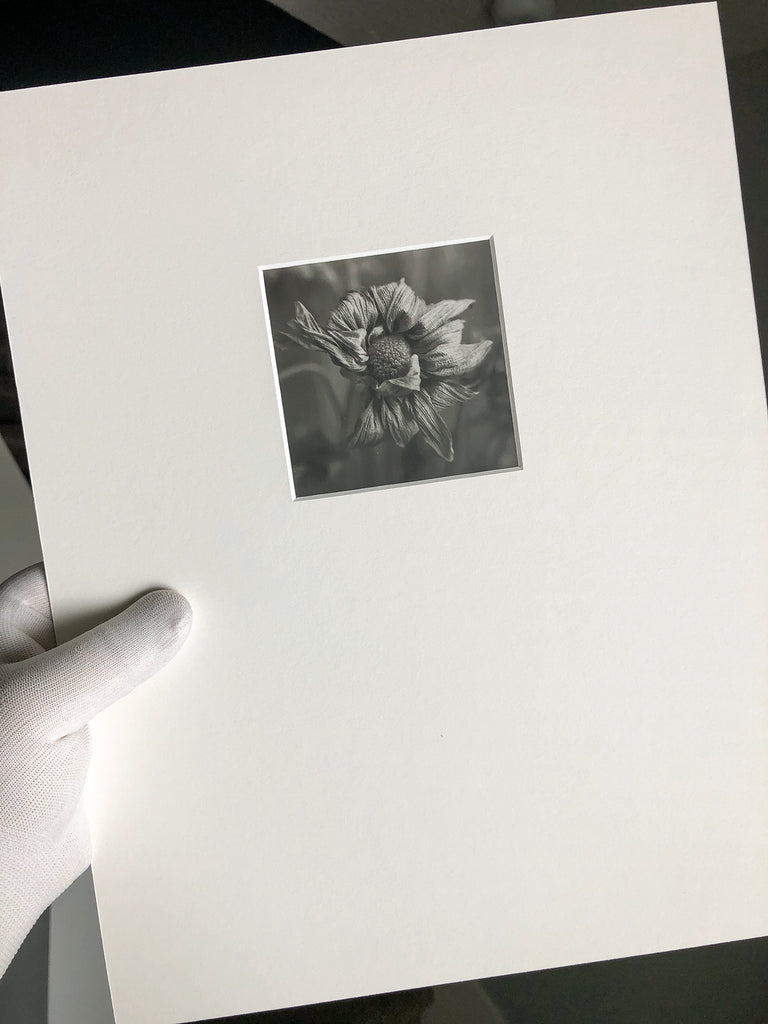The image is a detailed black and white photograph showing a close-up of a gloved hand. The hand, wearing what appears to be a white fabric glove, reaches in from the lower left corner, exhibiting a textured, unnatural appearance due to the glove. It holds a vertically rectangular, white piece of matting, akin to a standard sheet of paper, without any borders. This matting frames a smaller, centrally positioned square black and white image, approximately four by four inches. The square image inside the mat features a slightly faded, wilting flower, possibly a daisy, with sparse details but visible petals and a darker center. The background of the overall frame is notably white, contrasting with the dark and undefined backdrop that fills the upper left, right, and lower right corners, accentuating the starkness of the flower's black and white depiction.